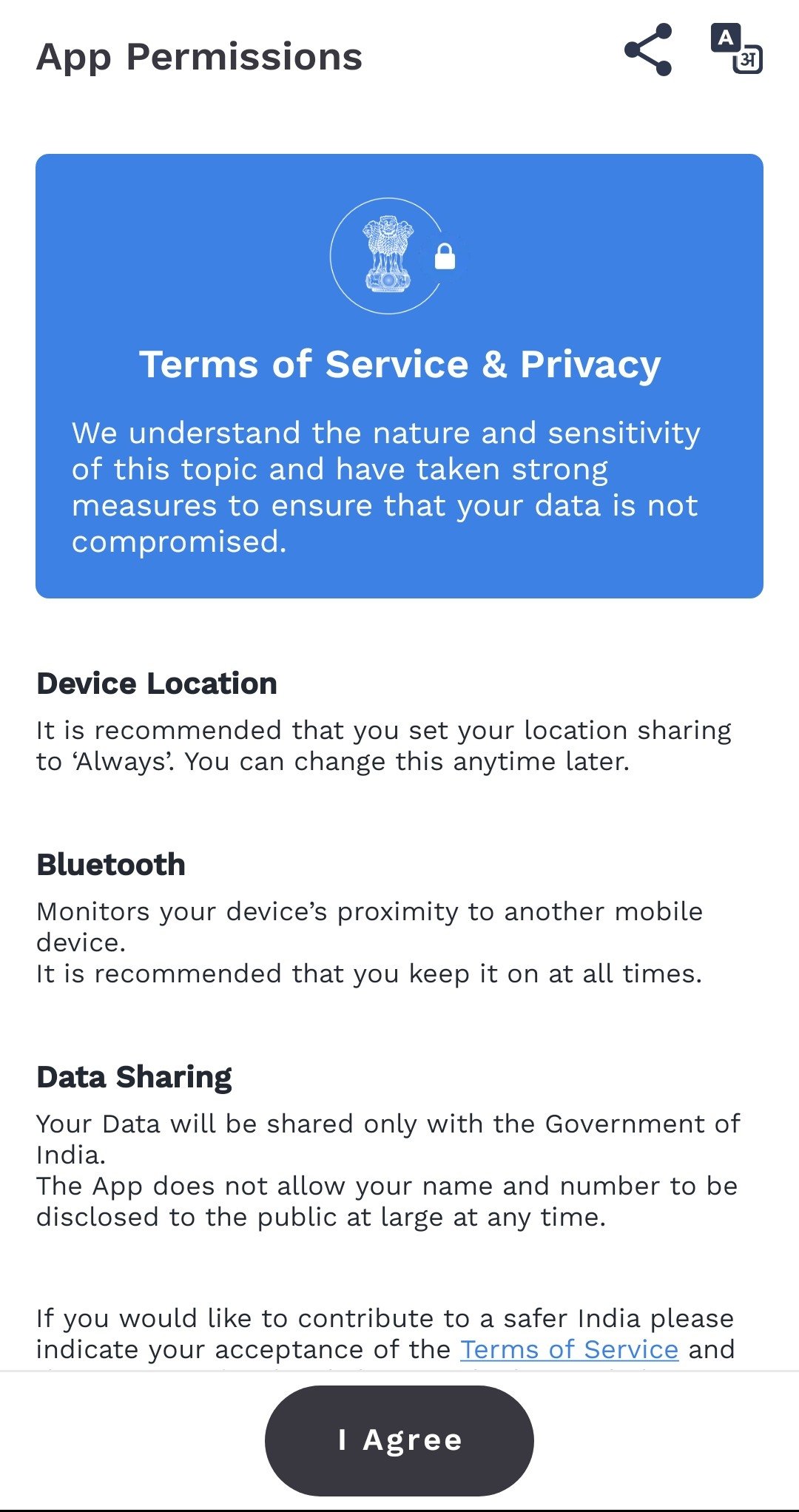Title: Privacy and Data Sharing Consent Page

Caption:

The image displays a user consent page with a mix of text and graphical elements, designed to ensure the privacy and data security of the user. At the top left corner, there's a black square containing the letter "A". Below it, housed within a blue box, are the words "Terms of Service and Privacy" in white letters, emphasizing the importance of user consent and data protection.

Following this, a detailed statement in white text reads: "We understand the nature and sensitivity of this topic and that they've taken a strong measure to ensure your data is not compromised." This reassures the user of stringent data security measures.

Beneath, in black letters, four key points are listed:

1. **Device Location:** Recommended for sharing always for undisclosed reasons.
2. **Bluetooth Data Sharing:** Monitors your device's proximity to other devices.
3. **Data Sharing:** Data will only be shared with the government of India, ensuring that no personal identifiers such as name or number are released to the public.

At the bottom of these points, there is a black circle containing the words "I Agree" in white letters, inviting the user to give their consent. A black line runs along the bottom, adding visual separation.

In a final note, a sentence encourages patriotic participation: "If you'd like to contribute to a safer India, please indicate your acceptance of the Terms of Services." The phrase "Terms of Services" is highlighted in blue letters, making it a clickable link for further details.